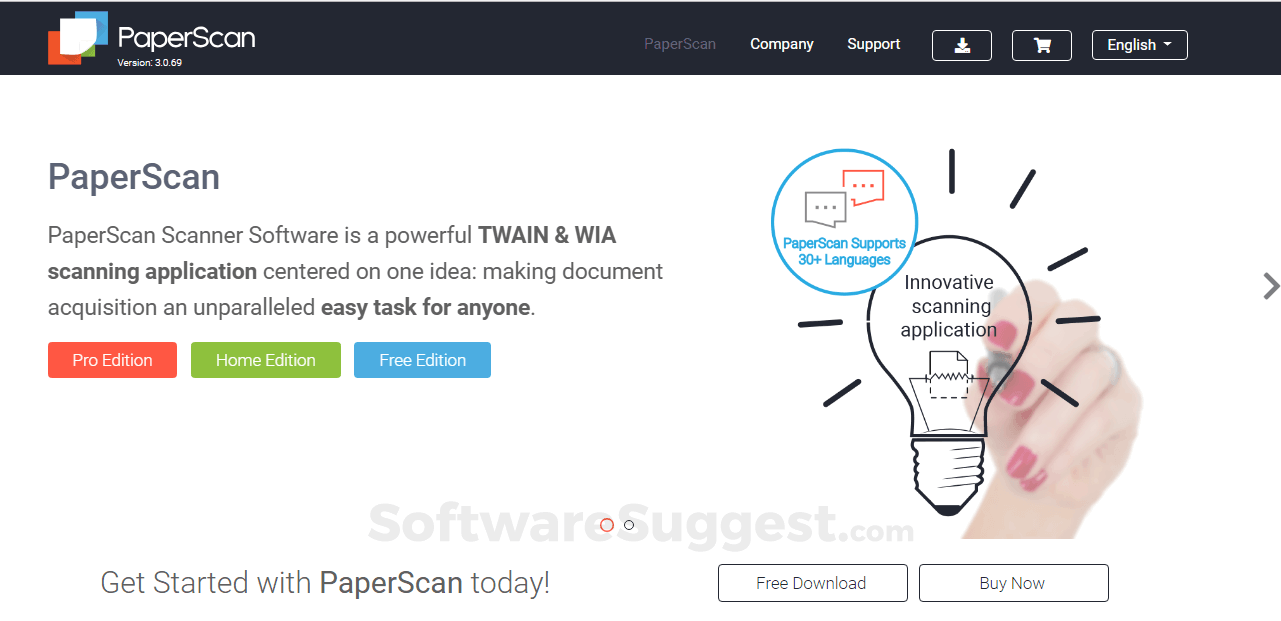The advertisement for Paper Scan is a rectangular landscape, approximately twice as wide as it is high. Across the top, there's a thin black rectangle running along the top border. In the upper left corner, "Paper Scan" is written in white, with both 'P' and 'S' capitalized. Beneath it, in a smaller font, the version number is displayed as either "3.0.59" or something similar. The Paper Scan logo, positioned to the left of the text, features three squares arranged in a somewhat triangular pattern, colored red, white, and light blue, with the white square overlapping the other two.

To the right of this black bar are clickable sections labeled "Company" and "Support." Further right, there are icons indicating a download, a shopping cart, and a language selection option labeled "English" with a small down arrow for changing the language settings.

The bulk of the advertisement is set against a white or possibly light gray background. The center of the ad repeats "Paper Scan" and includes three lines of descriptive text, highlighting that Paper Scan's scanner software is a robust TWAIN and WIA application focused on a singular idea.

Below this description are three horizontally oriented colored rectangles representing different editions of the software: a red rectangle for the Pro Edition, a green rectangle for the Home Edition, and a light blue rectangle for the Free Edition.

To the right, an illustration features a woman's hand with red nail polish holding a pen, drawing a light bulb from behind. The light bulb has lines emanating from it, signifying that it is lit. A light blue circle to the upper left of the bulb proclaims that Paper Scan supports "30+ languages."

At the bottom right, two rectangular buttons offer options for "Free Download" and "Buy Now," with both buttons being longer than they are high. In the lower left corner, floating text encourages viewers to "Get Started with Paper Scan Today."

Overall, the ad is a visually rich and detailed promotion, clearly designed to inform viewers about the features and editions of Paper Scan, and to encourage both downloads and purchases.